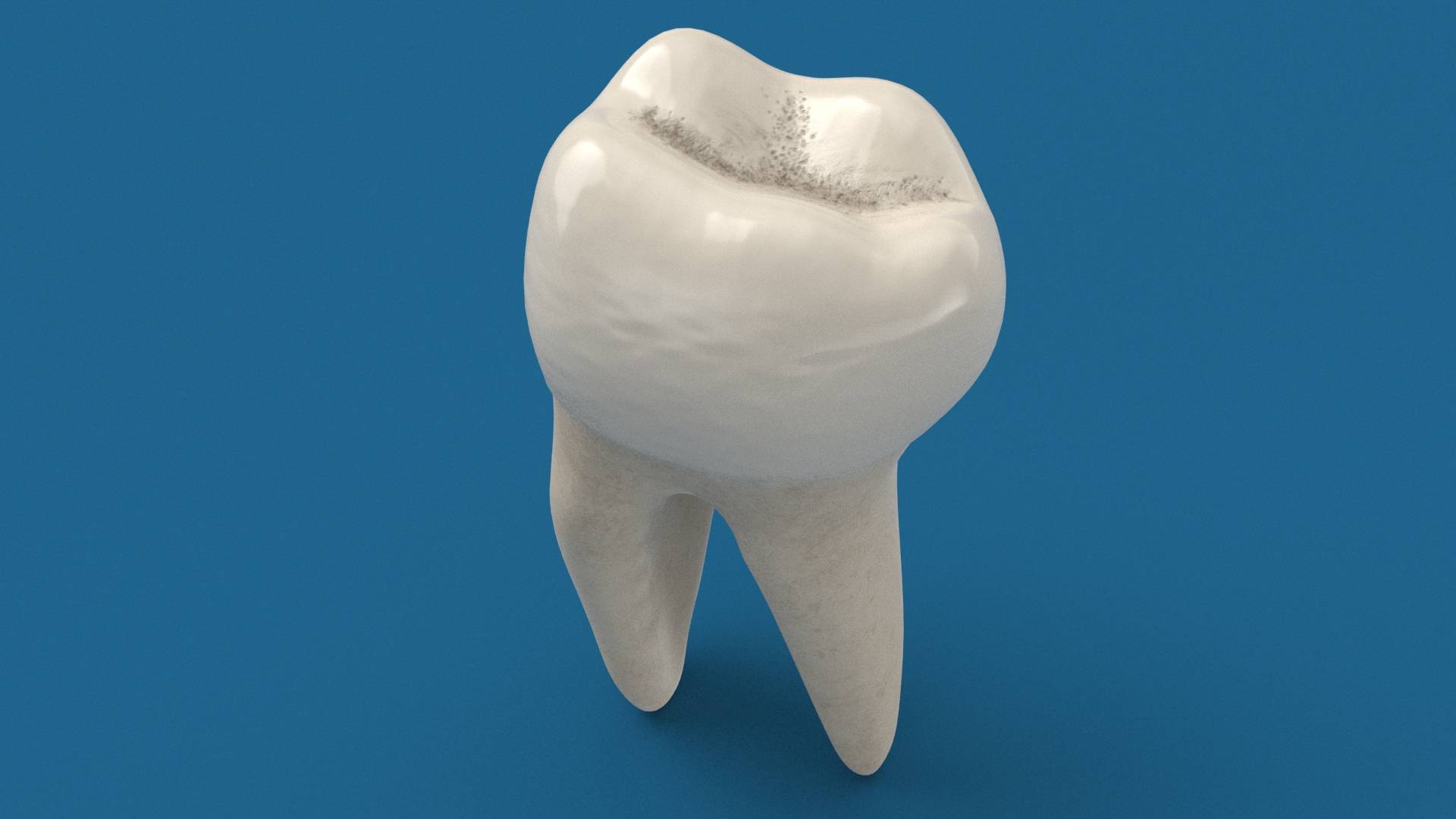The image presents a computer-generated depiction of a single white tooth set against a darker blue rectangular background. The tooth stands upright on two root-like points, slightly angling to the right, giving the appearance of legs. The surface of the tooth has a glossy, ceramic-like quality with a creamy white color at the top that transitions into a more beige-white at the bottom. There's a hollow point in the middle of these two supporting roots. The top of the tooth has noticeable indents and grooves that house numerous small black specks, contributing to a dirty or worn look. Light reflects off the upper left corner of the tooth, highlighting its texture and uniformity, which suggests it is an artificial representation rather than a real tooth. Shadows cast by the tooth and within its grooves add depth to the image.